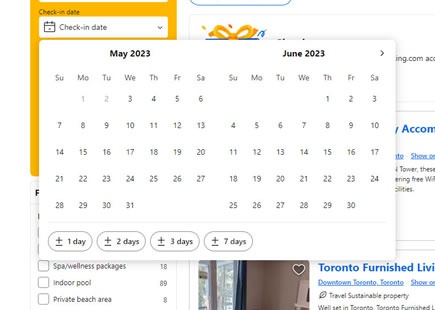The image displays a webpage prominently featuring a golden rod-colored square at the top. This square contains the text "Check-In Date" in white, accompanied by a dropdown menu. Below this, there are multiple options accompanied by checkboxes. Although the top part is obscured, the visible options read: "Spa/Wellness Package $18", "Indoor Pool $89", and "Private Beach Area $8."

Another section on the website, partially hidden by a large pop-up calendar, reveals more banners and choices. The calendar itself spans two months: May 2023 and June 2023, displaying their respective dates. At the bottom of the image, within the calendar pop-up, are four selectable options labeled with different date ranges: "+/- 1 day," "+/- 2 days," "+/- 3 days," and "+/- 7 days." The underlying webpage appears to be for "Toronto Furnished Living," although this is partially obscured by the calendar overlay.